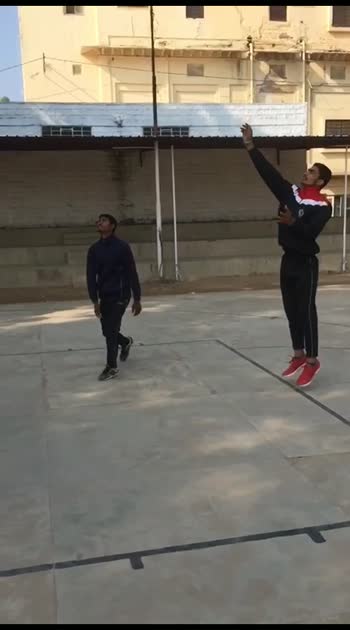In the image, two young men are playing basketball on an outdoor sports court. The player on the right is captured mid-jump, with his right arm extended as if he has just taken a shot from the three-point line. He is dressed in a tracksuit featuring a black base with red and white accents, including a red collar and red sneakers. The other young man, clad in a completely black outfit with dark shoes, is partially crouched and watching the trajectory of the unseen basketball. The basketball hoop is not visible in the frame. The background includes multiple layered buildings in shades of yellow, beige, white, and brown, along with a tan structure featuring an awning bordering the court. The court itself appears to be made of concrete, marked with black tape to delineate different sections. There is no text in the photo.